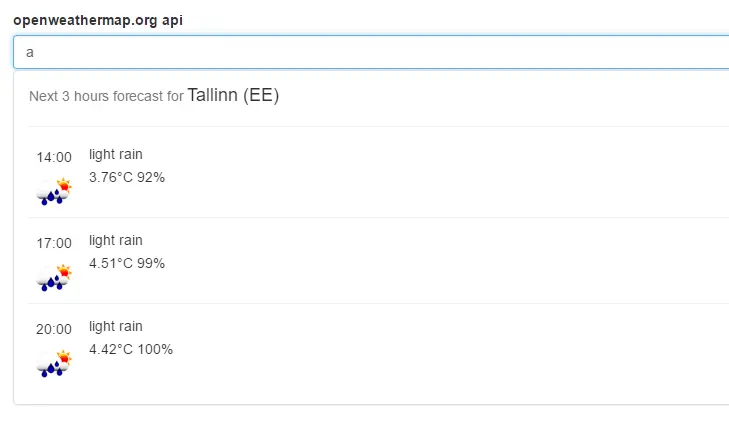This is a detailed description of a screenshot from a website or app, specifically from the OpenWeatherMap API at openweathermap.org. The image has a predominantly white background and is oriented horizontally. Most of the content is aligned to the left side, leaving a significant amount of blank space on the right.

At the top of the screenshot, the website address "openweathermap.org API" is displayed in bold. Below it is an open text box with a blue border, partially cut off on the right side. The text box appears to be designed for user input, with an "A" typed into it.

Following the text box, there's a section titled "Next Three Hours Forecast for Tallinn," written as "T-a-l-l-i-n-e-e." The forecast breakdown is as follows:

- At 1400 hours, the weather is indicated as "light rain," with a temperature of 3.67 degrees Celsius and a 92% chance of rain. An icon representing rain with purple raindrops and a red sun accompanies this information.
- At 1700 hours, the forecast again predicts "light rain," with the same rain icon.
- At 2100 hours, "light rain" is also forecasted, with an updated chance of rain at 99% for the first time period and 100% for the second.

The icons and text are consistently placed, providing a streamlined view of the upcoming weather conditions for the specified location.